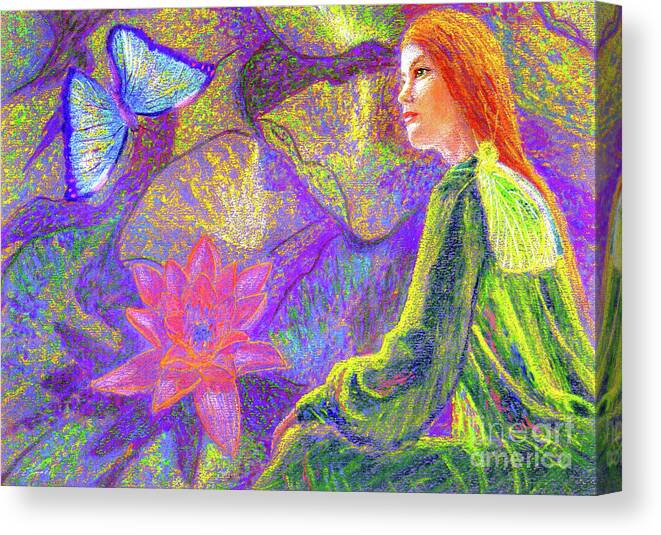The image is a vivid painting, possibly an oil or pastel piece, depicting a red-haired woman dressed in a long green dress sitting in a fantastical, abstract scene rich with plant life and vibrant colors. Her pale skin contrasts with her fiery hair, highlighted with streaks of yellow, and she gazes off to the left towards a blue butterfly fluttering in the upper left corner. A vibrant greenish-yellow insect, possibly a mayfly or lacewing, sits on her shoulder. The background is a blend of abstract purples with splashes of yellow, red, and green, creating an otherworldly atmosphere. Below the butterfly, there's a red lotus-like flower, and the overall ambience suggests she might be a goddess of plants or life. The painting is marked with a subtle watermark at the bottom right, indicating it might be sourced from In Art America.